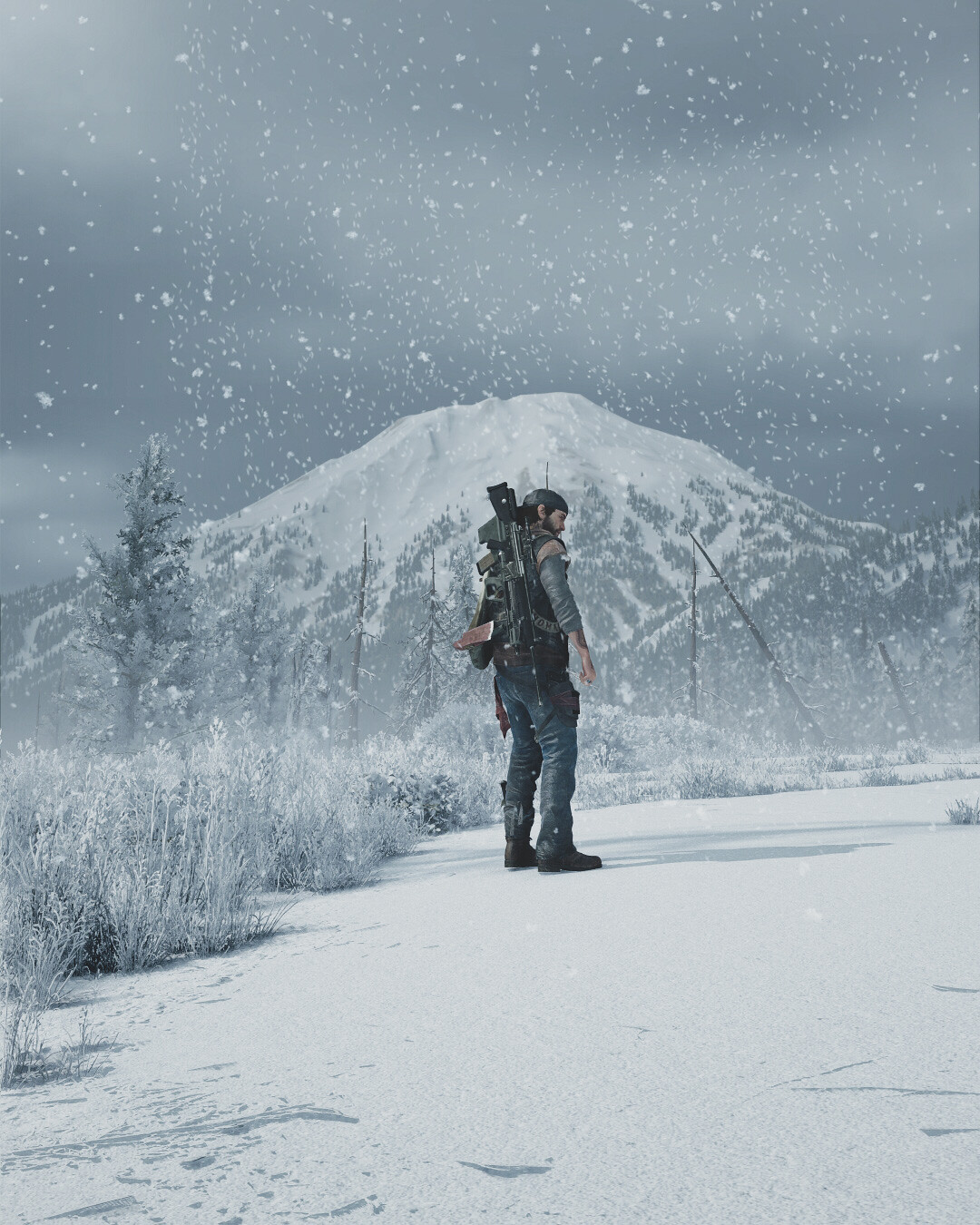This image, which appears to be either a screen grab from a video game or a computer-generated drawing, depicts a rugged individual standing ready for combat. The character is outfitted with military gear, including a large rifle strapped to his back, combat-ready pants, and sturdy boots. He sports a backward ball cap and a blackish-brown beard, suggesting a seasoned fighter. The scene is set in a snowy, mountainous landscape. Snowflakes fall gently around him, blanketing the mountain's peak in white. To his left, bushes and trees provide rough terrain, while his shadow stretches out to the right. The sky in the background is a hazy blend of snowflakes, adding to the wintry atmosphere.